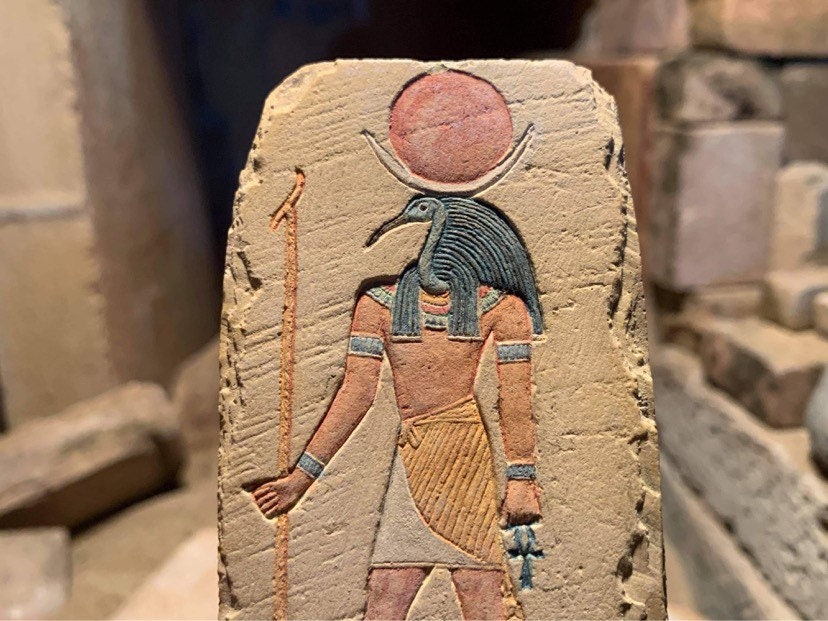This photograph captures a close-up view of an ancient Egyptian artifact, meticulously etched on a rectangular stone that appears aged and chipped around the edges. In the center of the image stands an intricately carved hieroglyphic depicting a humanoid figure adorned in traditional Egyptian attire. The figure sports a bird-like head with bluish-green feathers flowing back like hair, representing what looks like a swan. Above the head sits a distinctive arc cradling a red sun, symbolizing Ra. The figure is clad in a gold and white cloth wrap around the waist, accentuated by ornate wristbands, bands around the biceps, and a bluish-green collar around the neck. In its right hand, the figure holds a staff, while the left hand, pointing downward, grasps an ankh, an ancient Egyptian symbol of life. The background is blurred, giving a seamless impression of stacked stone blocks or similar artifacts, drawing our focus to the rich detailing of the primary hieroglyphic.